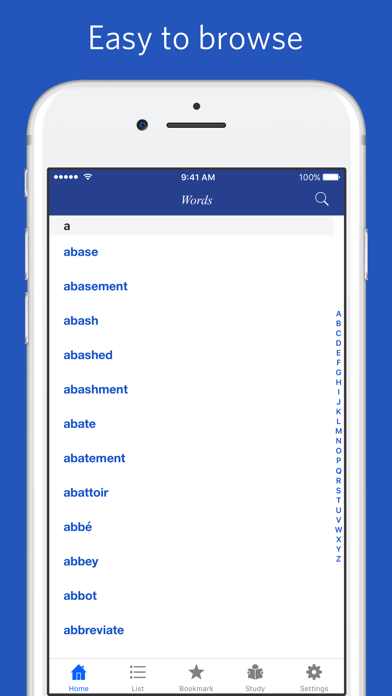The top portion of the image displays the text "Easy to Browse" in white, situated above a partial view of a cell phone's interface. This interface includes the status bar, showing the time as 9:41 a.m. to the left, and a fully charged battery icon on the right. Below the status bar is a search bar with a magnifying glass icon on the right, labeled "words."

The main content starts with a line of text displaying a lowercase "a." Following this, there is a vertical list of words, each separated by about an inch and a half of space. The words listed are: 
- abase (a-b-a-s-e)
- abasement (a-b-a-s-e-m-e-n-t)
- abash (a-b-a-s-h)
- abashed (a-b-a-s-h-e-d)
- abashment (a-b-a-s-h-m-e-n-t)
- abate (a-b-a-t-e)
- abatement (a-b-a-t-e-m-e-n-t)
- abattoir (a-b-a-t-t-o-i-r)
- abbé (a-b-b-é)
- abbey (a-b-b-e-y)
- abet (a-b-e-t)
- abbot (a-b-b-o-t)
- abbreviate (a-b-b-r-e-v-i-a-t-e)

At the base of the image, the phone's navigation options are visible. These options include: Home, List, Bookmark, Study, and Settings.